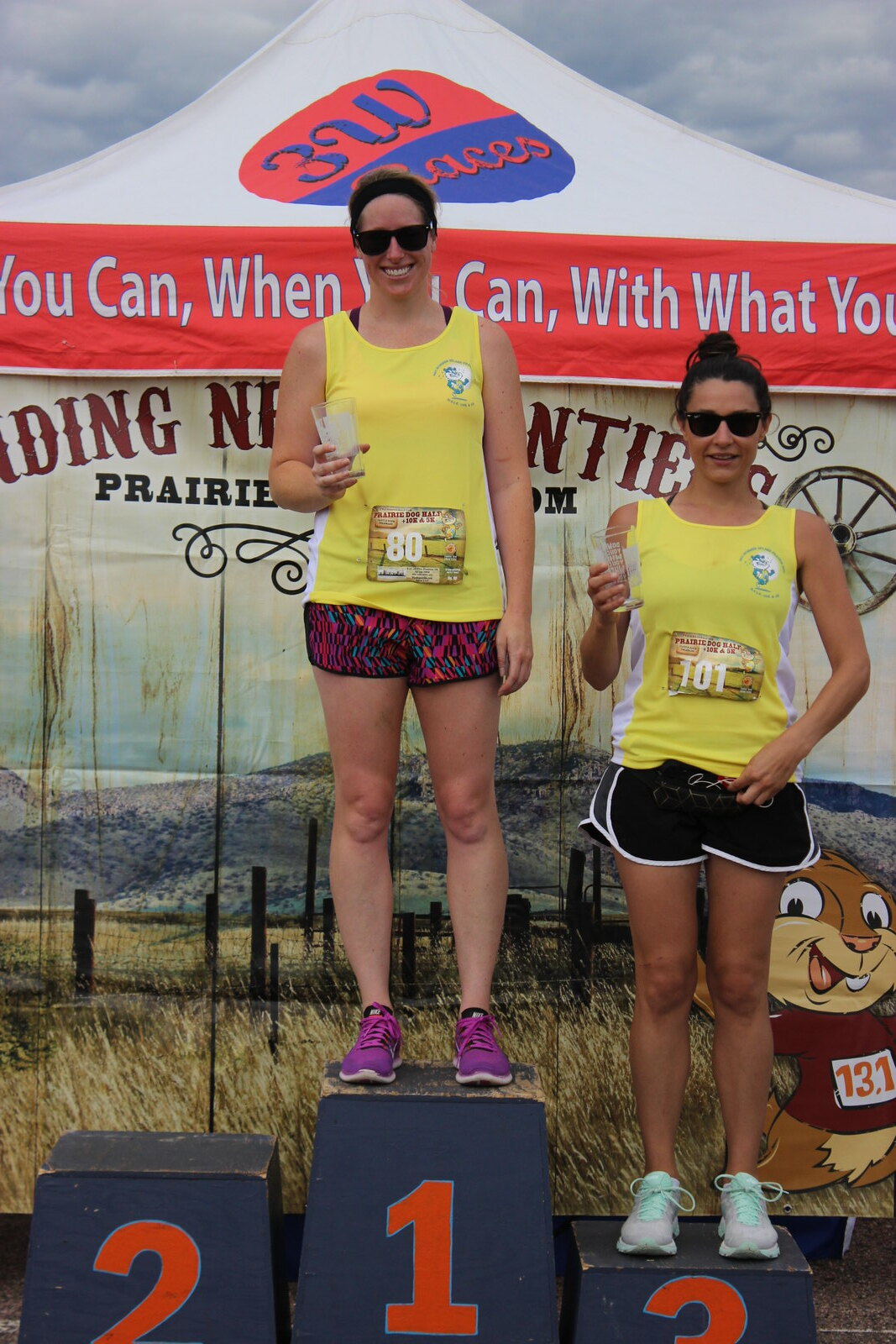A vibrant photograph captures two women standing on winners' platforms, beaming with pride. The woman on the highest platform, labeled "1," signifies her first-place victory, while the second woman stands on the third-place platform, labeled "3." The second-place platform remains vacant. Behind them, a backdrop resembling a tent displays partially visible motivational text, "You can where you can with what you." Both women are clad in matching yellow tank tops and are accessorized with sunglasses. They hold ornate glass trophies, possibly made of crystal, presumably awarded for their achievements. Their radiant smiles and direct gaze at the camera reflect their joy and accomplishment. The ground beneath them is not clearly visible, reinforcing the focus on their triumph. This scene clearly marks their impressive finishes in a race.